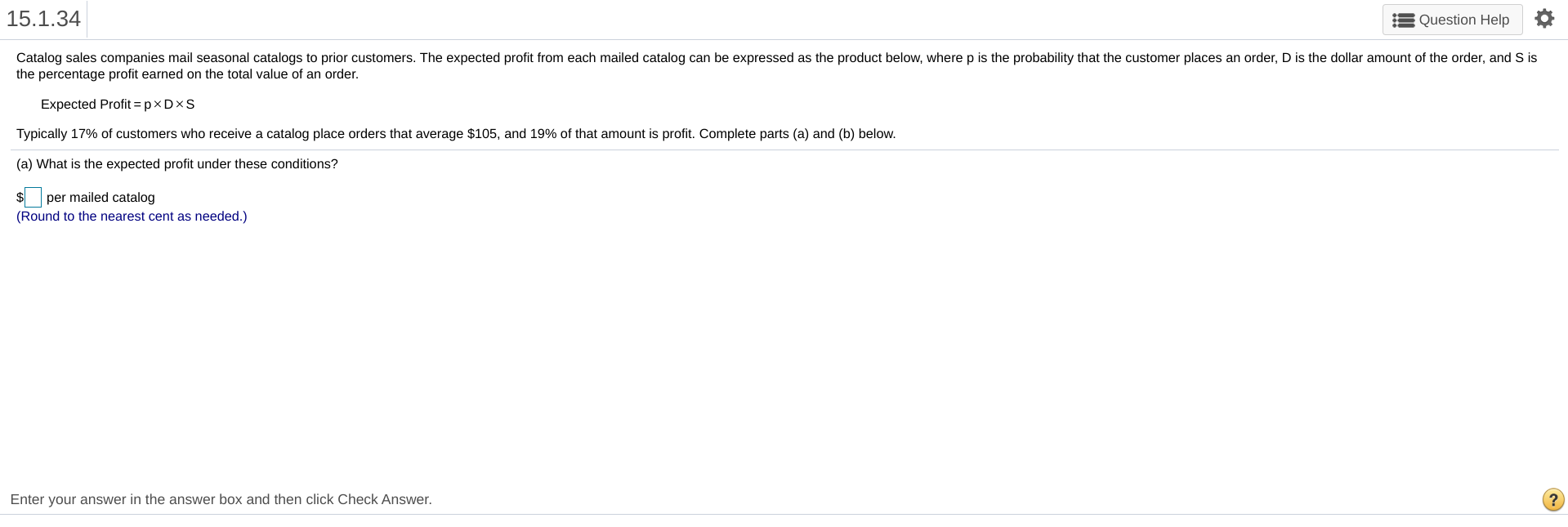The image depicts a low-resolution screen capture from a device, characterized by its pixelated and blurry quality. At the top left corner, the screen displays the code "15.1.34." On the top right, a button labeled "Question, Help" is visible alongside a settings icon. Below this, the text starts on the left with several categories listed: "Catalog," "Sales," "Companies," "Mail," and "Seasonal Catalogs To Prior Customers." The description continues to explain that the expected profit from each mail catalog can be calculated using the formula: expected profit = P x D x S. Here, "P" stands for the probability that a customer places an order, "D" represents the dollar amount of the order, and "S" signifies the percentage profit earned on the total value of the order.